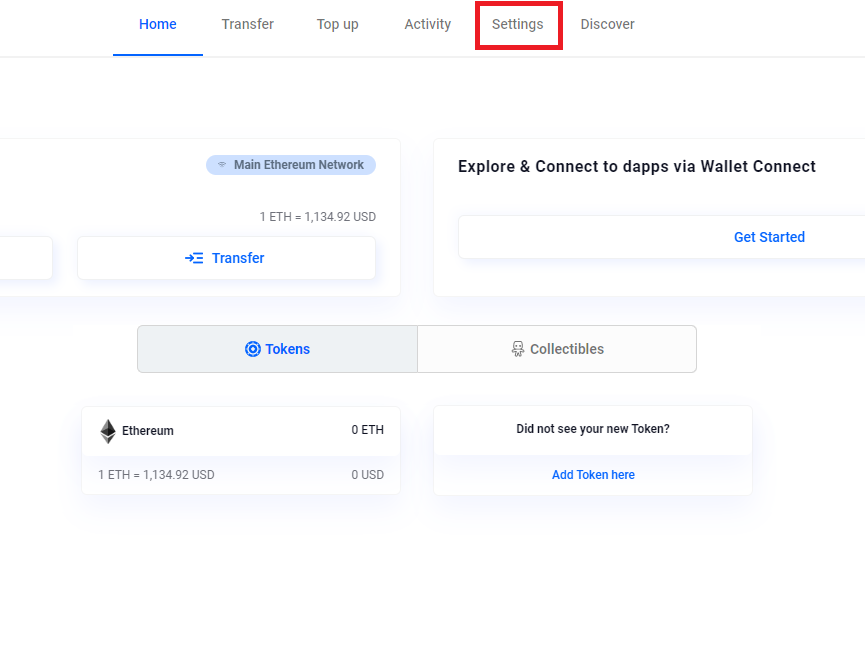The screenshot displays a computer screen featuring a comprehensive dashboard layout. At the top, there's a navigation bar with six categories: "Home" (underlined), "Transfer," "Top Up," "Cat Activity," and "Settings" (highlighted in a white box with a red outline), followed by "Discover."

Below the navigation bar is a white box displaying information about the Main Ethereum Network, highlighting that 1 Ethereum equals $1134.92 USD.

Further down, there's another white box with "Transfer" in blue text. Next to it is another section that reads "Explore and connect to DAPPs via WalletConnect," followed by a blue "Get Started" button in a white rectangular box.

The subsequent row features the headings "Token" (in blue text) and "Collectibles" (in gray text). Below this, the Ethereum symbol (a diamond) appears with the label "Ethereum" and "0 ETH" underneath it. This is accompanied by the reiterated rate of 1 Ethereum equaling $1134.92 USD.

Lastly, another column displays the message "Did not see your new token" beneath the previous row.